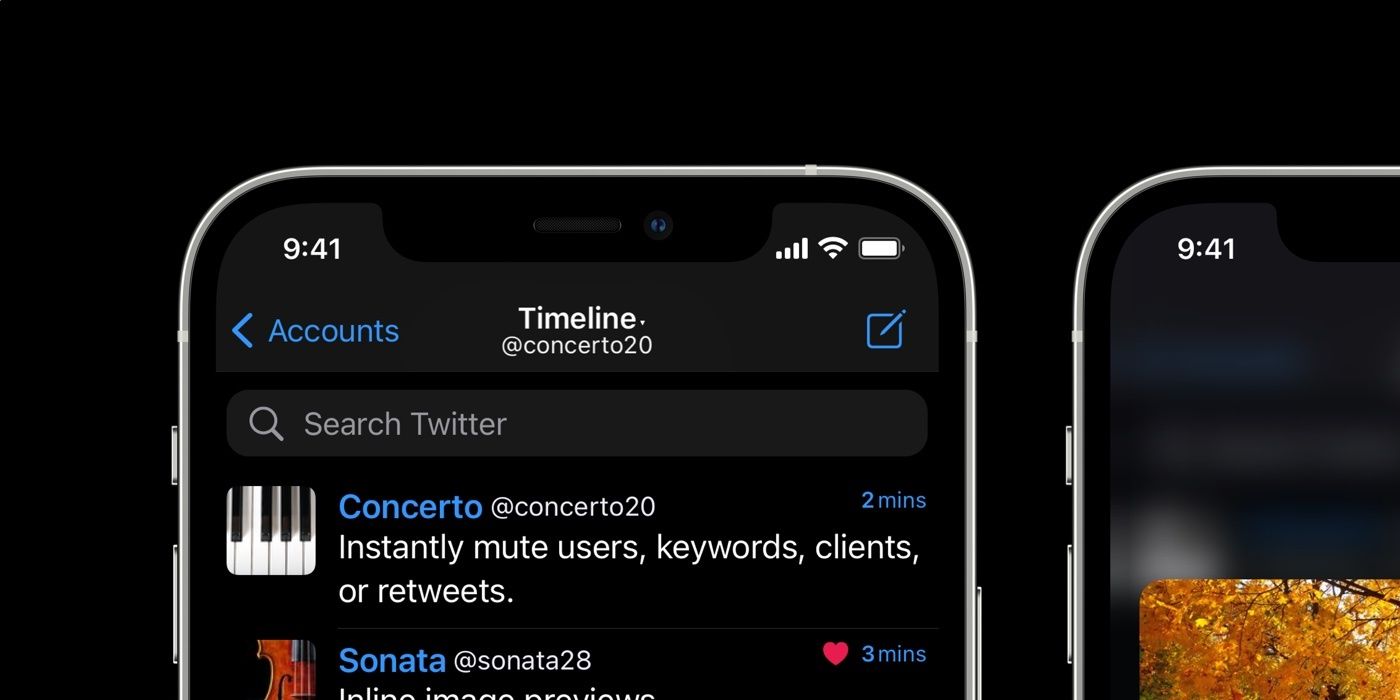Detailed Caption:

The image displays a smartphone interface with a dark theme. At the top left corner, the time reads 9:41, alongside the mobile signal strength icon, Wi-Fi icon, and a full battery indicator. Dominating the screen, the word "Timeline" is prominently centered in white text. Below the search bar, which has the text "Search Twitter" typed in it, there is an interaction list. The text "CONCERTO" and the handle "@CONCERTO20" are highlighted in blue, followed by the phrase "Instantly mute users, keywords, clients, or retweets," which was done in two minutes, also highlighted in blue. An icon resembling piano keys is situated beside "CONCERTO."

Further down, "SONATA," with the handle "@SONATA28," is likewise highlighted in blue. Adjacent to this, a heart icon is visible, and the text "3 minutes" is highlighted in blue. A tiny picture of either a violin or bass instrument accompanies the "@SONATA28" handle. The backdrop of the interface is predominantly black, creating a striking contrast with the white and blue highlights.

The screen of another phone nearby shows a scenic image of autumn trees with bright yellow-orange leaves, suggesting daytime. This second phone also displays the time 9:41 at the upper left corner. Both screens together create a visual impression of an organized and user-friendly interface amidst a serene autumn setting.